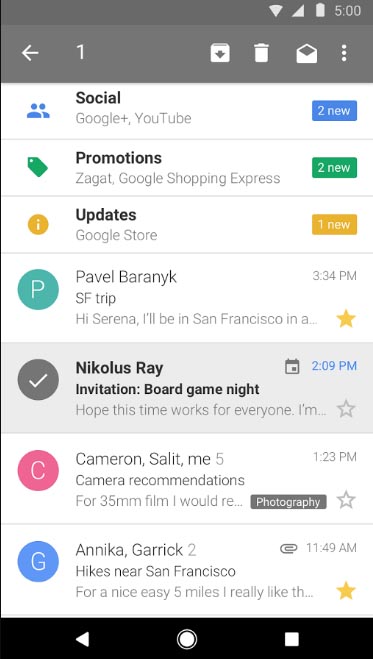A detailed screenshot of a cell phone email application is depicted, with a grey header at the top. On the left of this header, the number "1" is displayed followed by a left-pointing arrow. Four icons are arranged to the right: a box with a downward arrow in the center, an icon of a trash can, an envelope icon, and finally, a three-dots icon for additional options.

The body of the screenshot features a white background. Positioned at the top in bold, dark font is the word "Social," indicating the active email tab. Directly below, it shows "Google YouTube," along with the label "2 new" enclosed in a green box on the right, signifying two new unread emails in this section. Beneath this, the "Promotions" folder is visible with another green box showing "2 new." Further down, the "Updates" folder is noted with a yellow box reading "1 new" to indicate one new unread email in this section.

The emails themselves are listed below these folders. The second email in this list is highlighted in grey and marked with a checkmark to the left, indicating that it has been selected.